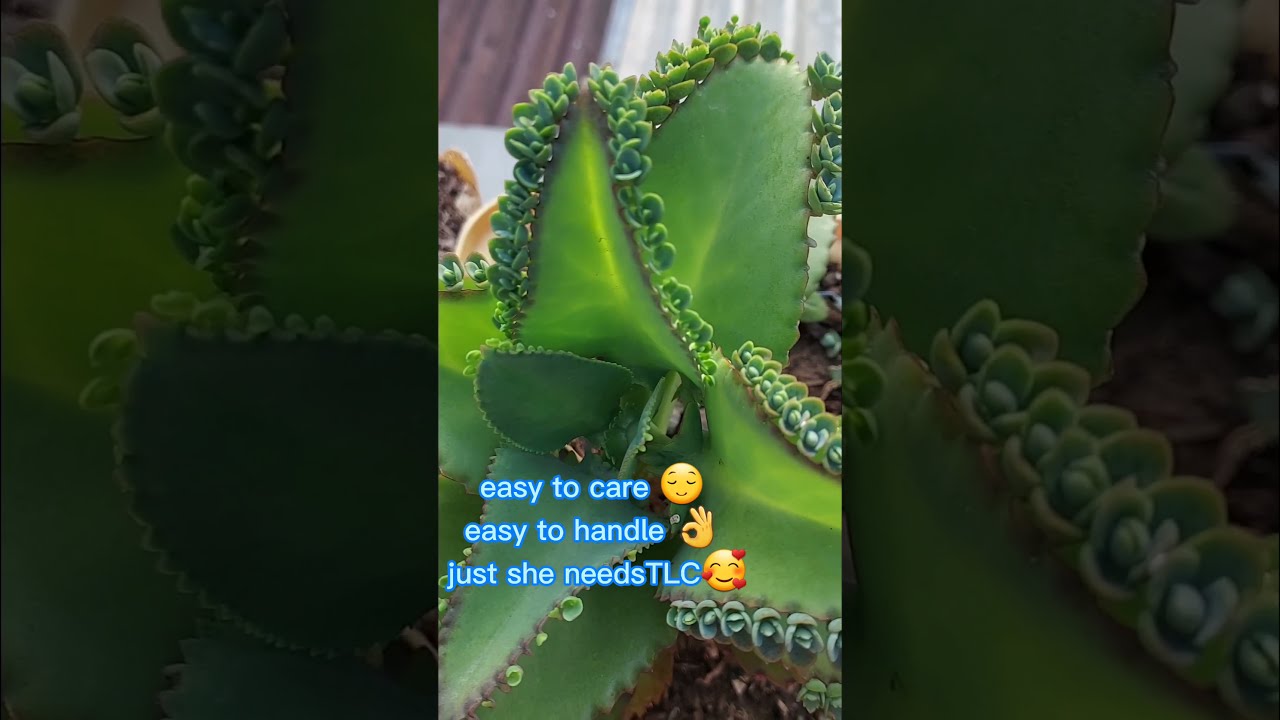The image is presented in a horizontal triangular box composed of three panels. The left and right panels are dark with green vegetation, while the central panel is lighter and more detailed. The central panel looks like an artistic rendition, possibly from a cartoon or video game, featuring a close-up of a lush, vibrant plant akin to an agave with thick, starfish-shaped leaves and tiny plantlets budding along the edges. The leaves exhibit a gradient from lighter green at the center to darker green at the edges. Overlaid on this image is text in white letters with a blue outline, stating: "Easy to Care" accompanied by a smiley face emoji, "Easy to Handle" next to a hand making an OK sign emoji, and "Just She Needs TLC" followed by a smiling face emoji with two hearts. Each of the three textual lines is emphasized by an adjacent emoji. The composition is framed by zoomed-in, faded-out background images of the same plant, enhancing the main photo's vividness and detail.